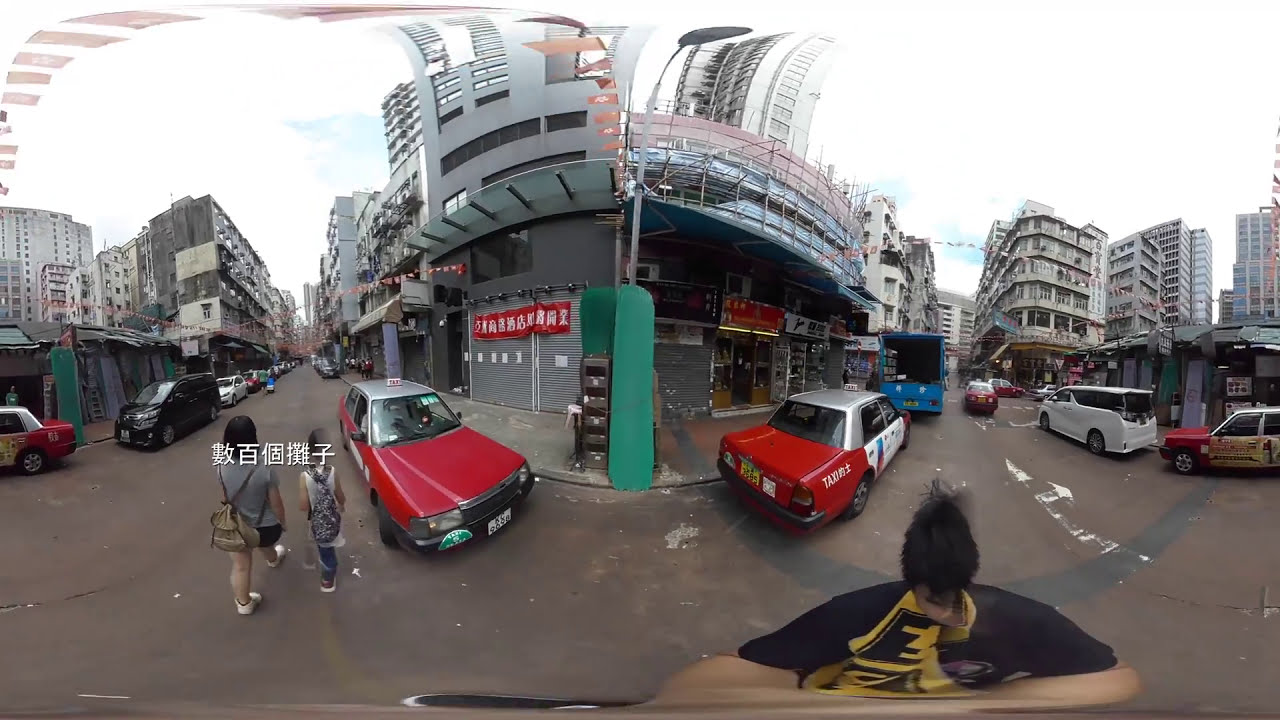The photograph captures a bustling, somewhat rundown city street in an Asian urban setting, likely an inner city area rather than a business or tourist district. The image appears to be a panoramic shot, which causes the buildings and street to bend and curve. Several red taxis dominate the foreground, along with a blue bus positioned to the right. Buildings, many of which are under construction, line both sides of the street, characterized by their gray, structured appearance and intricate elements. The asphalt road is filled with parked and moving cars, with a person riding a scooter visible. Two people, including a woman and a child, can be seen walking along the street but their figures are slightly distorted and their backs face the viewer. The sky overhead is overcast and gray, adding to the overall dreary atmosphere. Chinese characters are superimposed on the left side of the photograph, adding to the sense of place. The dominant color palette includes gray, yellow, black, brown, red, blue, orange, and silver, with a patch of white stretching across the top of the image, likely representing the cloudy sky.